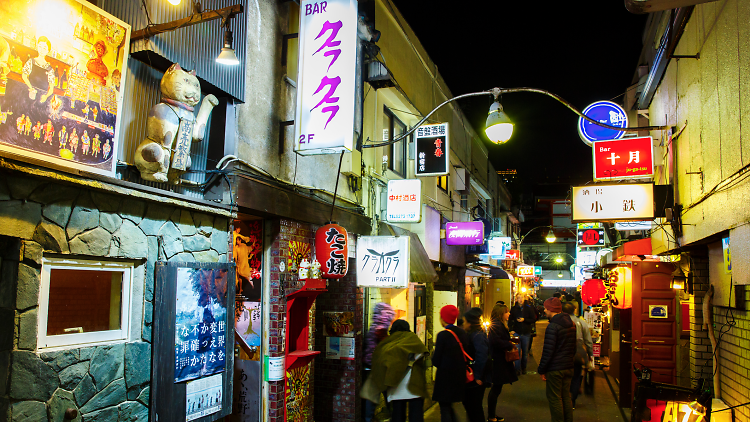This photograph depicts a bustling, narrow alleyway in an Asian market, possibly in Japan or China. Illuminated by overhead street lights that cast a warm yellow glow, the scene takes place at night, contributing to an intimate, cozy atmosphere. The alleyway is lined with small businesses and eateries, such as bars and ramen shops, with enough room for only 4 to 5 people to walk comfortably side by side. 

On the right side, a white brick building with a solid white second floor features multiple backlit signs with Asian characters. The signs, arranged vertically, include a blue circle at the top, a red square in the middle, and a white rectangle at the bottom. A red door in this building stands open, inviting passersby inside. Across the narrow street, the building on the bottom left corner has a facade resembling a mosaic of gray cobblestones, complete with a wooden signboard and a white-framed window. 

Further adding to the charm, cat statues adorn some of the shops, and the street is festooned with signage and small lights stretching overhead. People, both locals and foreigners, mill about, exploring the various businesses that remain open, possibly operating 24 hours. The alleyway, framed by taller structures in the distance, encapsulates the vibrant and eclectic essence of a busy Asian market street at night.